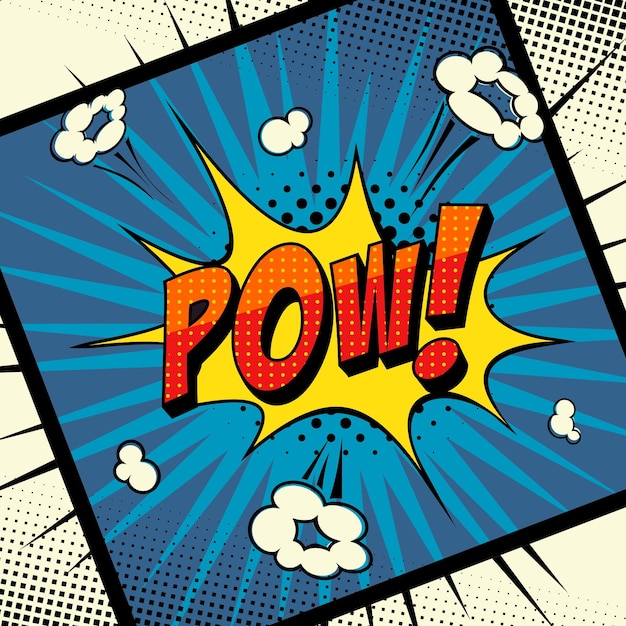This vibrant pop art style comic book image features the dynamic word "POW!" in bold orange letters with a gradient from light to dark orange, accented with white polka dots. The striking word is centrally positioned against a jagged, spiked yellow burst shape. Encircling this, smaller black dots add texture, while white, smoky cloud-like wisps radiate outward, enhancing the visual impact. Surrounding the yellow burst is a lighter blue, spiked bubble transitioning to a darker blue, framed by a diamond-shaped black square with jagged edges that extend into an off-white background peppered with black dots. The composition is intense and visually engaging, filled with contrasting colors like blue, yellow, orange, red, white, and black, typical of what you’d find in classic comic book art.